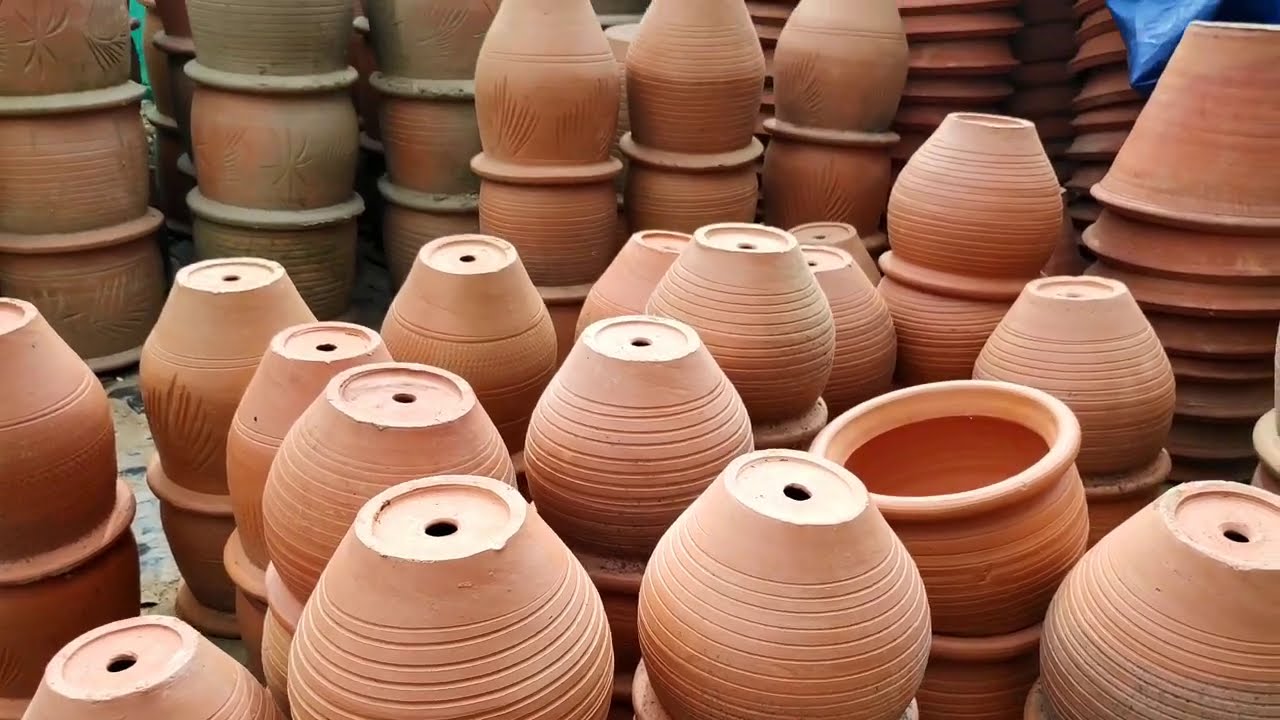The image showcases an arrangement of terracotta flower pots, predominantly tan and light brown. The vast majority are stacked upside down, while a couple are upright. The pots, which have a textured design as if etched with a rake while still malleable, dominate the frame. In the top right, a corner of a blue tarp is visible, possibly used for protection against moisture. The top left hints at a glimpse of aqua green between the pots, though the object is indeterminate. Concrete pavement is visible in the background, indicating the photo was likely taken outdoors, possibly in a garden center or the storage area of a home improvement store. The new pots in the foreground catch more light, highlighting their fresh, clean surfaces, while some pots in the rear show a greenish patina, suggesting weathering or age.